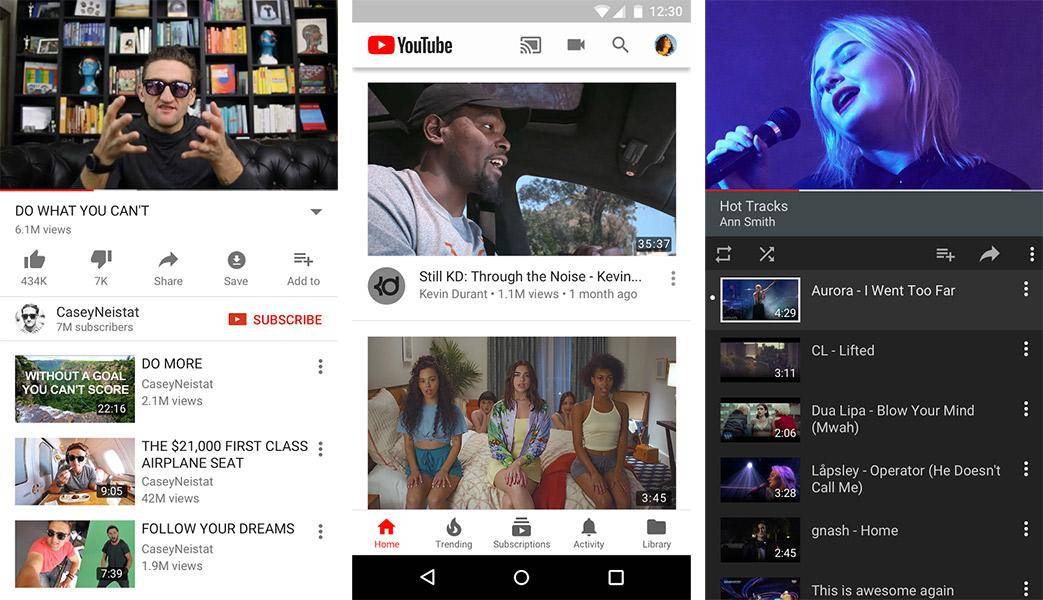The image depicts a YouTube homepage displayed on a computer screen at 12:30. Dominating the center are YouTube video previews. The first video, titled "Still KD Through the Noise," features Kevin Durant and was uploaded a month ago. Below this, there’s a thumbnail of three girls sitting on a bed, with two additional girls reclining.

The left sidebar highlights various options such as Home, Trending, Subscriptions, Activity, and Library. A featured video shows a man in sunglasses, presumably Casey Neistat, standing in front of a bookcase with the title "Do What You Can't," garnering 6.1 million views. Other visible videos in his section include "Do More Without a Goal You Can't Score," "First-Class Airplane Seat" showing him on a plane, and "Follow Your Dreams" depicting him in a seated stance.

On the right sidebar, under the section named "Hot Tracks," a track by Ann Smith titled "Aurora" is featured. Additionally, there’s a list of songs including "Lifted" by CL, "Blow Your Mind" by Dua Lipa, "Operator," and "Ganache." The last track is cut off but hints at the word "awesome."